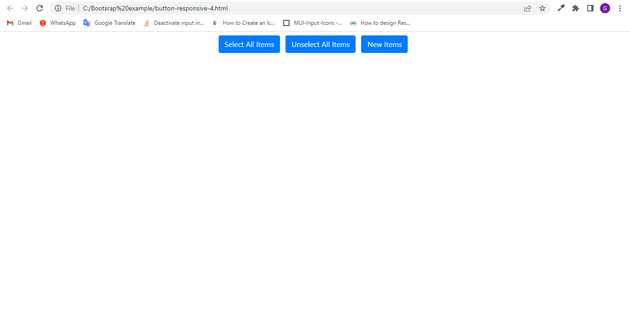This image showcases the top section of an internet browser window, capturing a detailed view that includes various browser interface elements and a blank web page with interactive buttons. 

At the very top of the image, on the browser's toolbars, viewers can observe the following elements from left to right:
- Forward and back navigation buttons, both represented by left and right arrows, which are grayed out, indicating they are non-functional at the moment.
- A refresh button for reloading the current webpage.
- The browser’s address bar, displaying a file path ending in ".html".
- Several icons to the right of the address bar, including:
  - A star icon, likely for bookmarking.
  - A puzzle piece icon, indicating browser extensions.
  - A purple circle with a letter inside, potentially representing the user's profile or account.
  - Three vertical dots, suggesting a menu for additional options.

Below this toolbar are quick access links to various websites, including Gmail, WhatsApp, Google Translate, and four other unspecified sites. 

Further down, just above the main content area, there are three prominently displayed blue buttons, arranged horizontally. These buttons are labeled as follows:
- "Select All Items"
- "Unselect All Items"
- "New Items"

The rest of the visible web page is completely blank, presenting a stark white background with no other content or elements.

The visual design details indicate that:
- The link bar is predominantly white, while the search bar has a slightly darker, grayish tone.
- The top navigation bar’s elements are clearly labeled and arranged for straightforward navigation and interaction.

This meticulous depiction suggests the image is intended to show a browser interface with fundamental navigation tools and a blank web page setup for further customization or action.